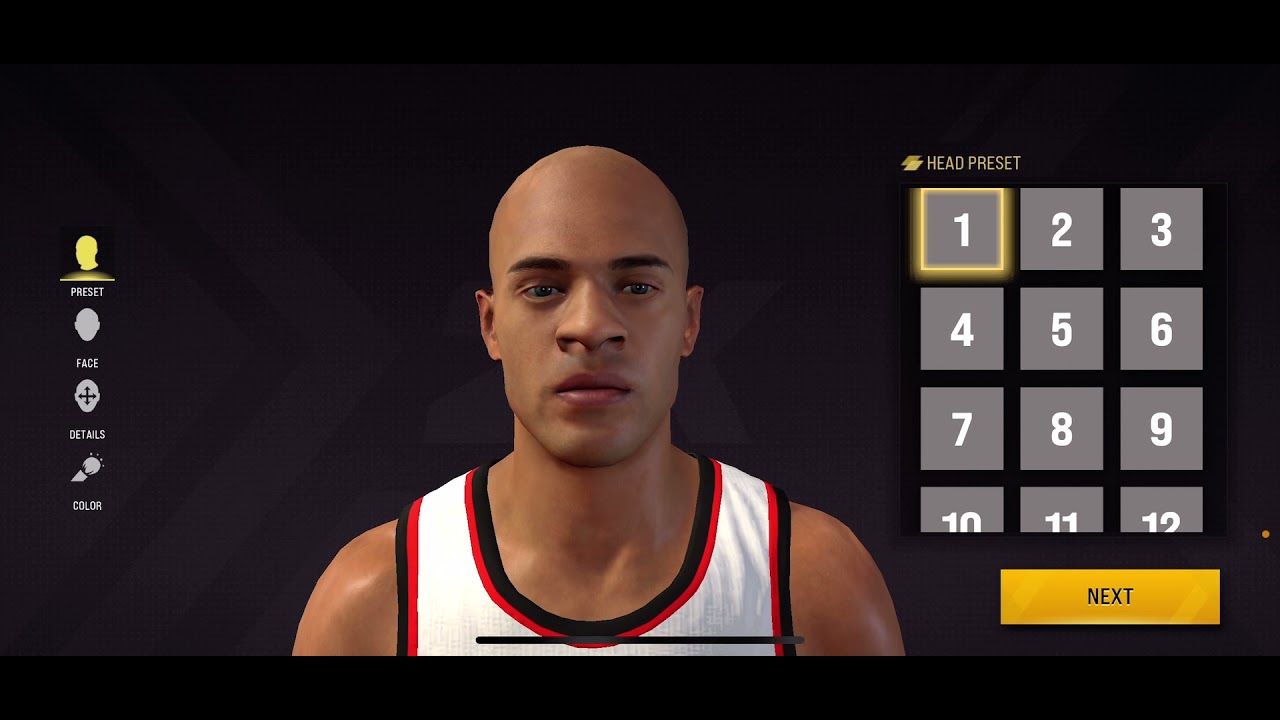The image appears to be a screenshot taken from a video game, depicting a character customization screen for a basketball player. The background is completely black, emphasizing the customization interface in the foreground. The character being edited is an African-American male wearing a predominantly white basketball jersey, accented with red and black trim. The man is bald, and the current selection appears to be focused on the "Head" options, as indicated by a highlighted tab.

On the left side of the screen, there are several customization categories listed vertically: "Preset," "Face," "Details," and "Color." The specific page displayed is the "Head Preset" section, which shows a grid of square options for different head presets. The grid is arranged in four rows, with each row containing three gray squares, each numbered in white text. The highlighted preset is '1,' distinguished by a yellow outline around the gray square.

Adjacent to the grid of presets, a "Next" button is prominently displayed in yellow, presumably to advance to additional customization options or presets.